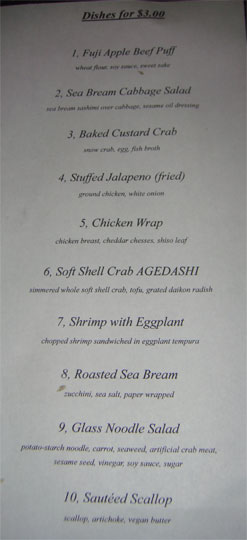In this vertically oriented photograph, captured on a mobile phone, we see a detailed menu printed on white paper. The menu, primarily written in italic font, lists 10 dishes, each priced at $3. Although the clarity of the image is not ideal, making some descriptions difficult to decipher, the main items are as follows:

1. **Fuji Apple Beef Puff:** Includes an unreadable description beneath it.
2. **Sea Bream Cabbage Salad:** The description is also unreadable.
3. **Baked Custard Crab:** Mention of "Snow Crab Egg Fish Broth?" but not fully legible.
4. **Stuffed Jalapeno** (without the ñ): Described as fried, containing ground chicken and white onion.
5. **Chicken Wrap:** Contains chicken breast, cheddar cheese, and another indistinguishable leaf ingredient.
6. **Soft Shell Crab Agedashi:** The term "AGEDASHI" is in capitals; it involves a whole soft shell crab with additional unreadable details.
7. **Shrimp with Eggplant:** Described as chopped shrimp sandwiched in eggplant tempura.
8. **Roasted Sea Bream:** Includes zucchini and sea salt, possibly wrapped in paper.
9. **Glass Noodle Salad:** Contains no starch noodles, carrot, seaweed, artificial crab meat, sesame seeds, vinegar, soy sauce, and possibly sugar.
10. **Sauteed Scallop:** Made with scallop, artichoke, and vegan butter.

Overall, the photograph's poor quality makes it challenging to read the finer details under each dish listing.